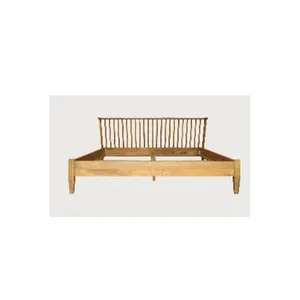The image depicts a simple, light pine wooden bed frame set against a light grey or off-white background. The frame itself features a headboard designed with vertical wooden slats arranged in a rectangular shape, providing a spindle-like appearance. The frame is devoid of any mattress, sheets, or pillows, highlighting its basic structure. The design includes a total of five legs: two at the front corners, two more at the back flanking the headboard, and one additional leg centered at the back for extra support. The bed frame is entirely constructed from wood, with no visible metal components. A middle support board runs from the headboard to the foot, ensuring stability for the mattress. Overall, the image captures a stark, minimalist, and functional bed frame.